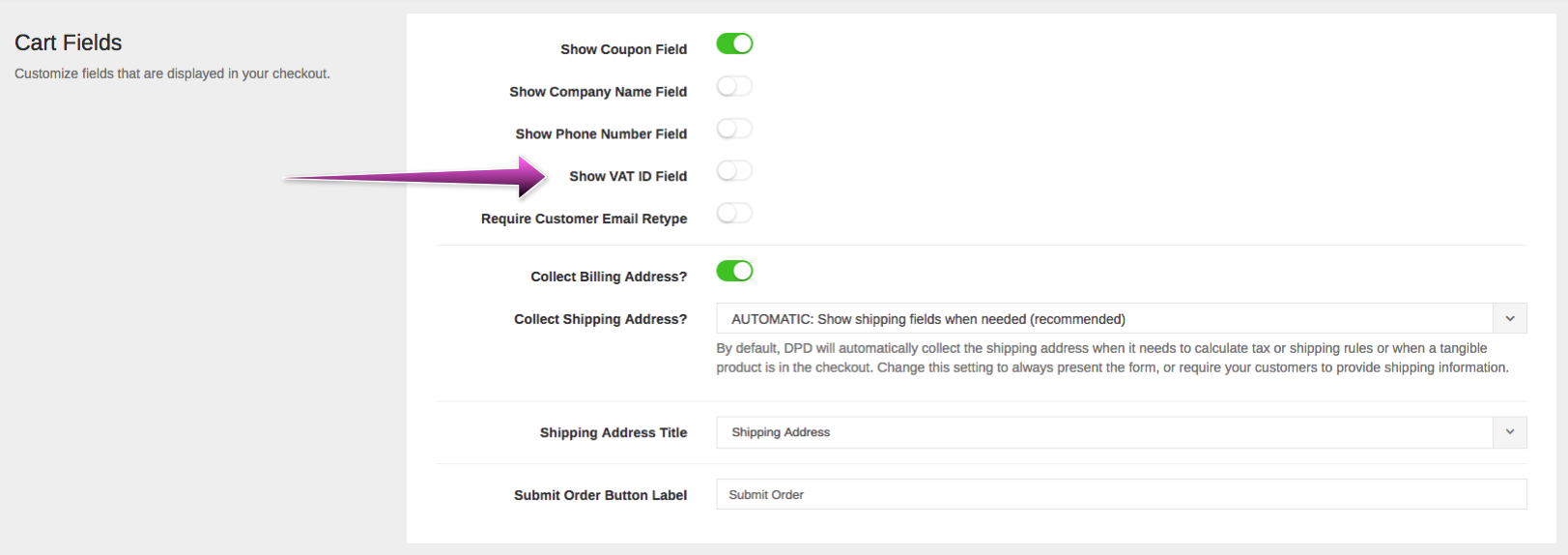The image displays a detailed interface for customizing the fields shown during checkout on an e-commerce platform. 

To the far left, the section titled "Cart Fields" is highlighted in black text. This section allows users to customize the fields that are displayed during the checkout process. The "Show Coupon Field" option is activated, indicated by a green toggle switch with a white circle positioned to the right. 

The "Show Company Name Field" option is inactive, with a plain white circle next to it. Other fields such as "Show Phone Number Field," "Show VAT ID Field," and "Require Customer Email Retype" are also listed. The "Show VAT ID Field" is distinctively marked with a purple arrow to the left. 

The "Collect Billing Address?" option appears with a toggle switch set to active, signifying that this option is turned on. Similarly, the "Collect Shipping Address Automatically" option is enabled by default, highlighted by a toggle switch moved to the right.

Below this, there is "Show Shipping Fields When Needed By Default" written in text, followed by "Shipping Address Title" in black text which provides the user with an input field to add their shipping address, indicated by a downward-pointing arrow inviting text input. 

At the bottom, there is a "Submit Order Button Label," and next to it, an area with an open box designed to input the order number before final submission.